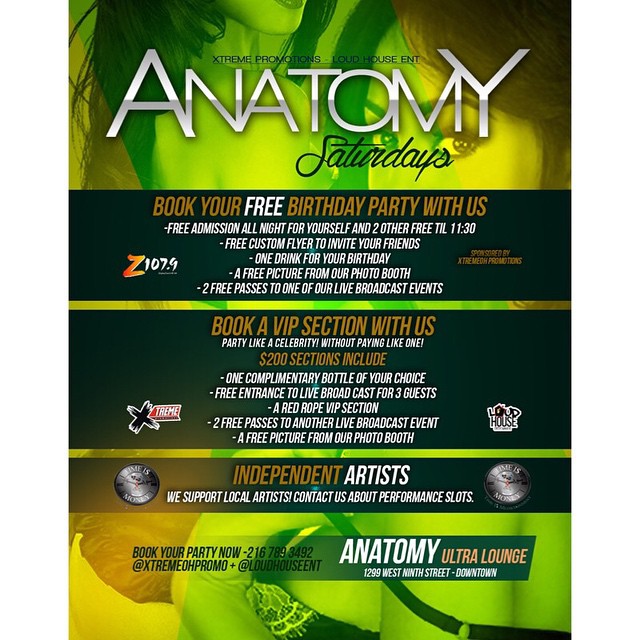This rectangular, portrait-oriented advertisement for Anatomy Ultra Lounge combines photographic elements with graphic design typography on a green and yellow tinted background. The photograph subtly showcases two scantily clothed women—one seen from a side profile and another with only the upper part of her face visible—dancing. 

Prominently positioned at the top is the headline "Anatomy Saturdays," with 'Anatomy' displayed in an all-white gradient and 'Saturdays' in a black script font. The center of the image features two horizontal black bands filled with yellow and white typography detailing various promotional offers. Key promotions include free birthday party bookings with offerings such as free admission for the celebrant and two others until 11:30 PM, a custom flyer to invite friends, one complimentary birthday drink, a picture from the photo booth, and two free passes to future live broadcast events. 

For a $200 VIP section, the package includes one complimentary bottle of choice, VIP red rope section entrance for three guests, and additional promotional benefits. The image also emphasizes support for local artists, inviting them to inquire about performance slots. 

The bottom band, also with a tint gradient, reads "Book Your Party Now" followed by contact details: 216-789-3492, Instagram handles @ExtremeOHPromo and @LoudHouseENT, and the venue address at 1299 West 9th Street, Downtown. The Z107.9 radio station logo is also prominently displayed, reinforcing the event's partnership. This comprehensive design effectively blends photographic and typographic elements to attract potential partygoers and highlight the venue's exclusive offerings.